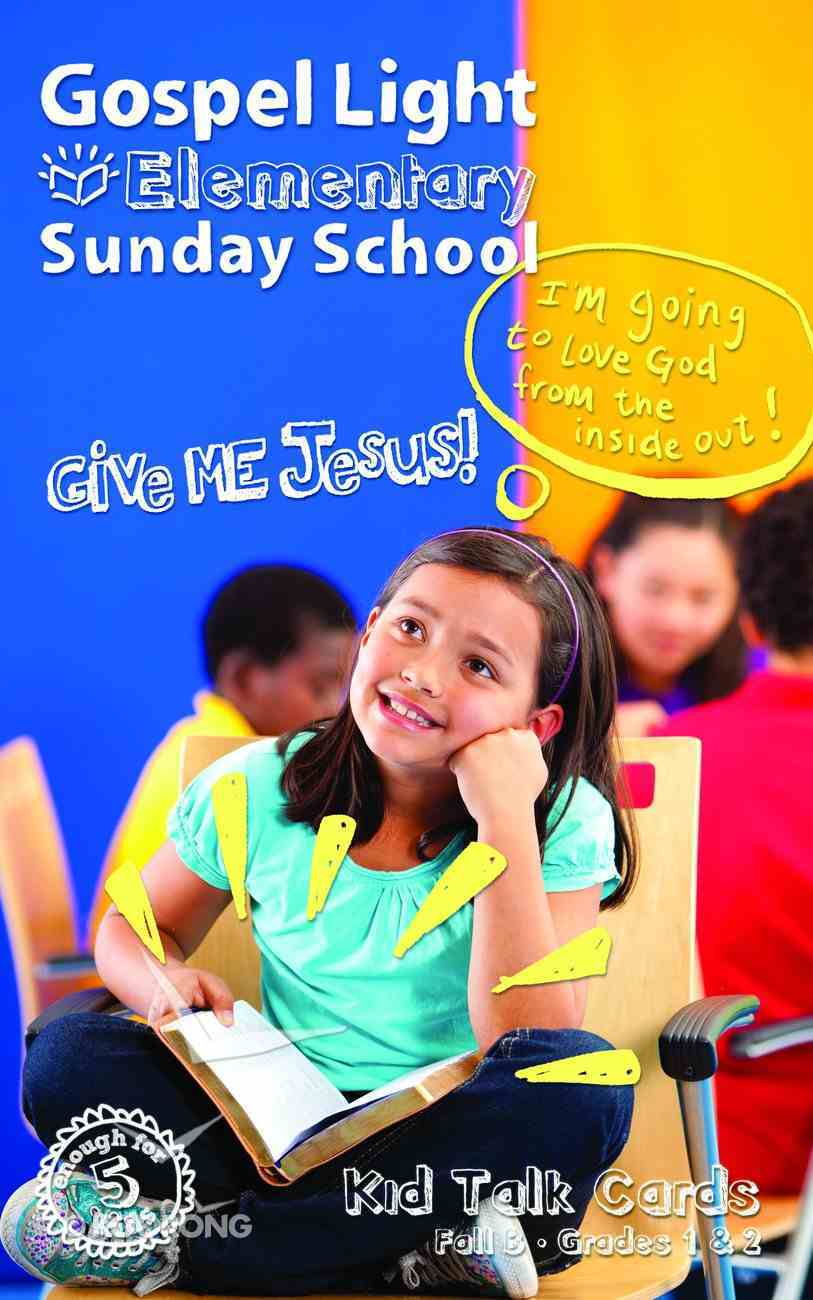The image is a colorful advertisement poster for Gospel Light Elementary Sunday School. Prominently, at the top left corner, it states "Gospel Light Elementary Sunday School" followed by "Give Me Jesus" in white text. The focal point of the image features a smiling girl with brown straight hair, dressed in a blue shirt. She is seated cross-legged, likely on a chair, with an open book, presumably the Bible, in front of her. Her left fist supports her cheek as she looks up thoughtfully. Positioned above her head is a yellow speech bubble that declares, "I'm going to love God from the inside out." In the background, there are blurred images of other children sitting in a circle on beige chairs. At the bottom of the poster, additional text highlights "Kid Talk Cards" along with references to fall grade levels 1 and 2. The scene is set inside what appears to be a classroom, filled with scattered colorful objects in hues of blue, pink, orange, yellow, purple, red, black, and brown.